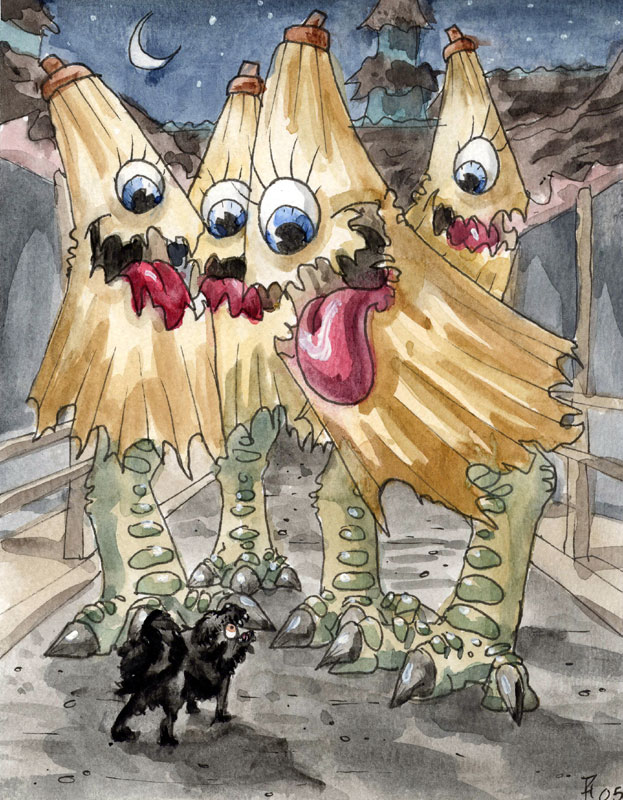In this surreal and detailed portrait-mode drawing, there are four bizarre creatures with tops resembling closed yellow umbrellas or the end of a banana peel. Each creature has a cyclopean eye with concentric circles of black, blue, and white and prominent eyelashes. Their mouths are open wide, showcasing large red tongues. The creatures' lower bodies feature green, reptilian legs with two toes, akin to dinosaur legs or dragon limbs.

The background reveals a deep blue night sky speckled with stars and a striking white crescent moon. These odd beings are positioned above what appears to be a bridge, indicated by the presence of railings on either side. 

Below these peculiar beings is a small black dog-like figure with a puffy tail and head, potentially having a nose or beak, which adds to its enigmatic appearance. The little creature is walking from the left towards the center of the frame and seems to be incredibly frightened, looking up at the surreal monsters above it. The artist's signature, resembling either Asian characters or a combination of the letters "P" and "H" along with the number "05," is inscribed in the bottom right-hand corner of the artwork.